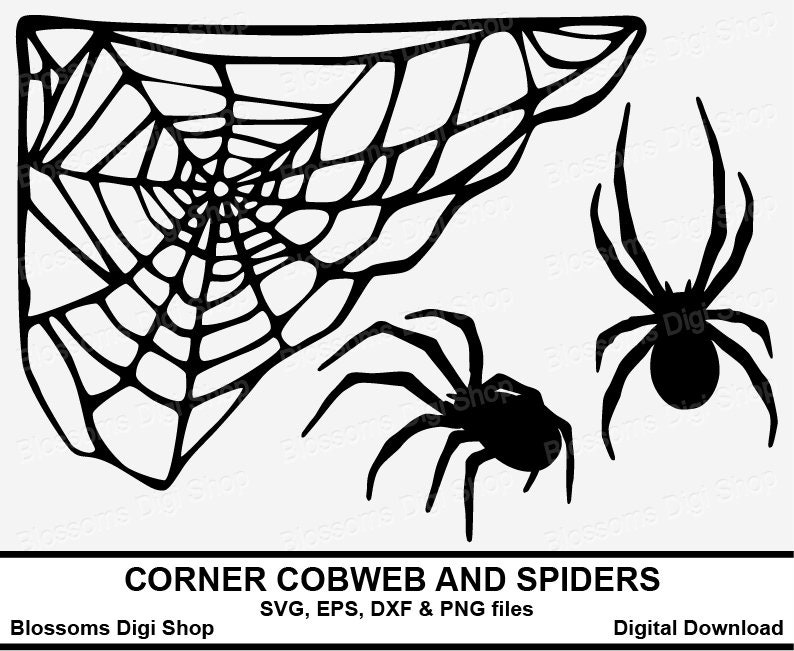The image is a white background depicting a digital download template from an online shop called Blossom DigiShop. It prominently features a large, triangular black spider web that occupies almost 40% of the space, extending diagonally from the bottom left to the top right. In addition, there are two drawn black spiders positioned to the right of the cobweb: the first spider is centrally placed and faces the top left toward the web, while the second spider is on the middle right, facing upwards. At the top of the image, there's a repeating watermark that reads "Blossom DigiShop."

Below the graphics, there are two horizontal black lines separating the image from the descriptive text. The first line of text reads "Corner Cobweb and Spiders," and the second line lists the available file formats: "SVG, EPS, DXF, and PNG files." At the lower left corner, the text states "Blossom DigiShop," and at the lower right corner, it says "Digital Download." All text and graphics are black on a white background, lending a minimalist yet informative aesthetic to the template designed for digital download purposes.